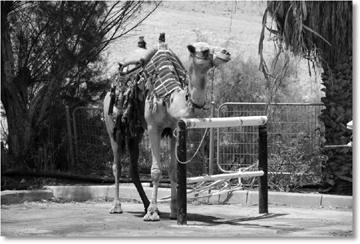This is a detailed, black and white photograph, featuring a camel as the central subject. Situated slightly to the left of center, the camel is facing towards the right in a diagonal orientation, making its front appear larger and closer. The camel is equipped with a blanket, possibly striped or plaid, and a saddle on its back. A rope is attached to its mouth and head, extending down to a white horizontal bar in front of it, which is supported by two vertical wooden poles on either side. The bar structure is reinforced by another white horizontal bar beneath the top one, connecting the two poles.

The setting appears to be a paved area, resembling a parking lot or street, with a curb visible in the image. Directly behind the camel is a metallic fence, about waist-high, with trees on the left and right sides of the image. Beyond the fencing, there are shrubs and grassy or hilly terrain, possibly sandy areas, but the exact nature of the landscape is indistinct due to the black and white nature of the photograph. The photo itself is a rectangle with slightly visible shadows along the right edge and bottom, giving it a photoshopped drop-shadow effect. The low resolution of the image adds to its antiquated charm.